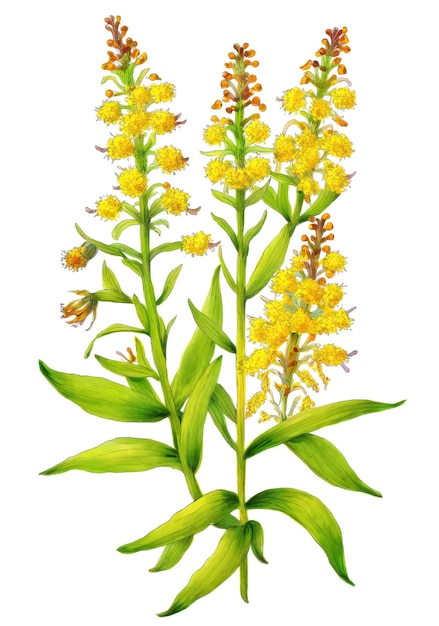This is a detailed color illustration of a flowering plant set against a white background. The plant features three tall, moderately thick stems adorned with narrow, sword-like leaves that are bright green, transitioning to a lime-yellow green hue. These leaves are oblong, pointy at the ends, and grow from both sides of the stalks. At the top of each stalk are clusters of extremely fluffy, pom-pom-like yellow flowers arranged in triangular shapes. Toward the top of these clusters are reddish-brown seed pods or buds, which appear poised to flower in the future. Additionally, some clusters have dead or shriveled flowers closed up around small green bases, possibly seed pods. The roots of the plant showcase these shriveled clusters and rich green leaves with dark to light green shades along the stem, giving a sense of natural growth and decay.